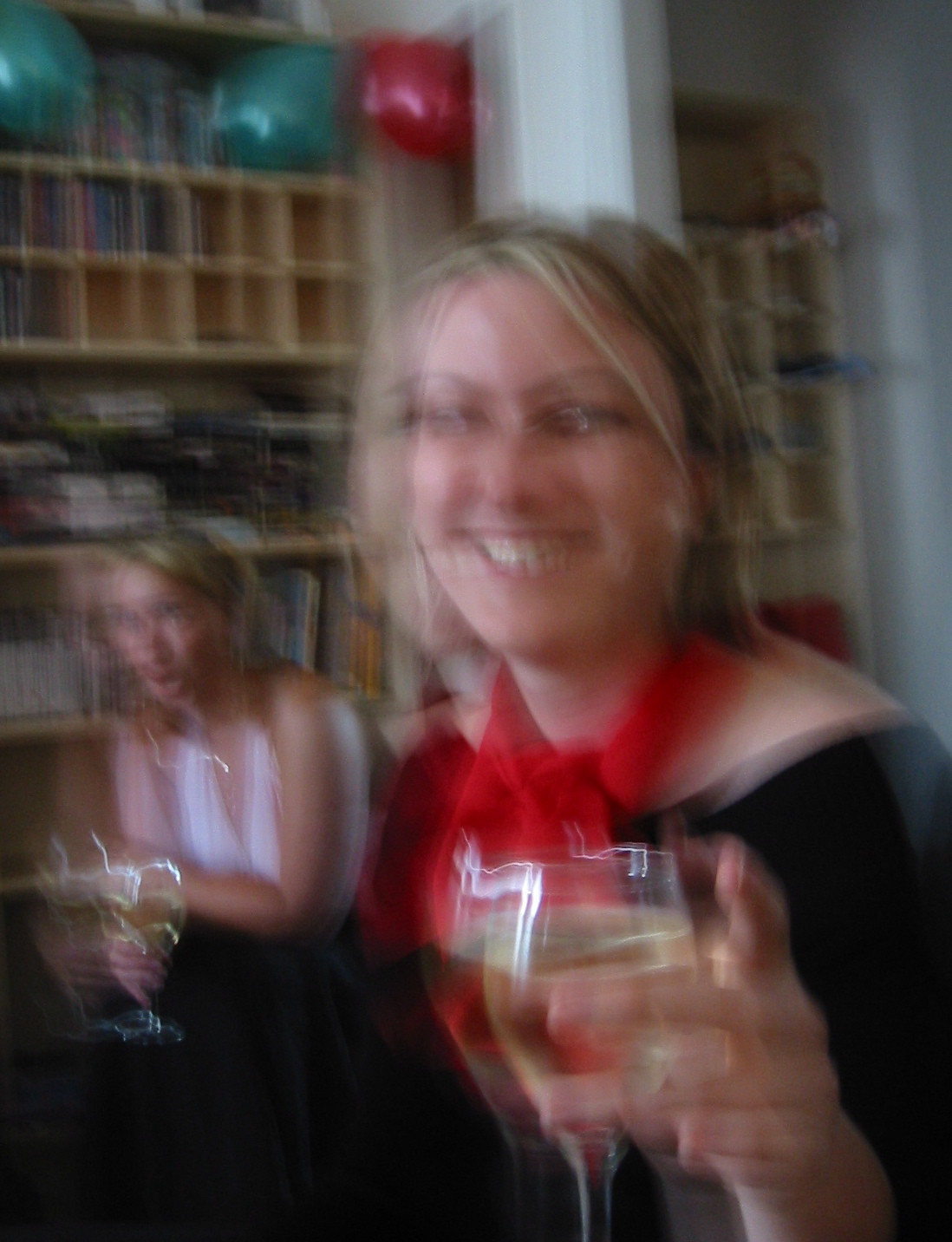This photograph, despite its blurriness, captures a joyous moment between two women at what appears to be a festive gathering, possibly a Christmas or birthday party. Both women are holding glasses of wine, exuding a celebratory spirit. 

The woman in the foreground, adorned in a black top and a vibrant red scarf, has blonde hair and is glowing with a broad smile. Her lively demeanor is complemented by the festive atmosphere. In the background, the second woman, also with blonde hair, is dressed in a white halter top paired with what seems to be a black skirt. Unlike her companion, she has a more neutral expression.

Behind them stands a white column, and to the side, shelves filled with books add a touch of coziness to the setting. Atop the shelves, several festive balloons—two green and one red—contribute to the celebratory decor, hinting at the party's cheerful theme.